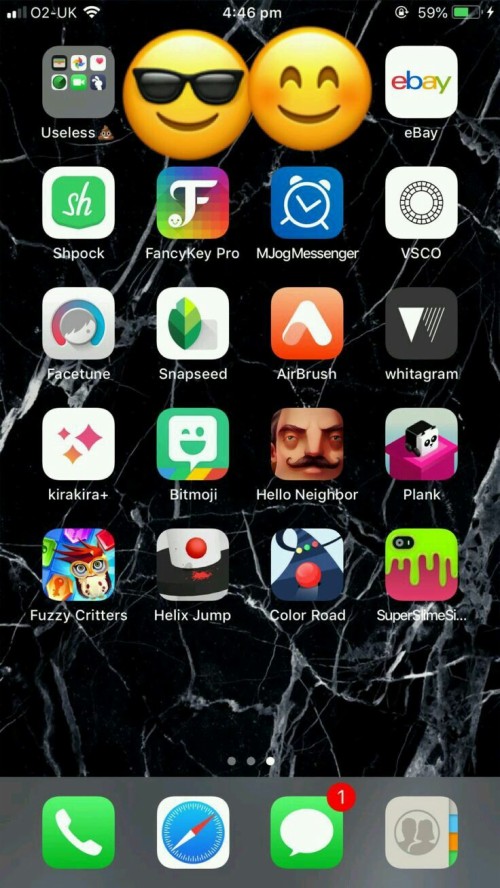Image Caption:

A sleek, black background is adorned with two expressive emojis—one wearing sunglasses and the other blushing. Within the frame, an image of a character named "Boo Boo" is prominently featured. The screen displays a plethora of apps, including eBay, Shpock, FancyKey Pro, Mjalk, Messenger, VSCO, FaceTime, Snapseed, AirBrush, Litagram, Kirakiri Plus, Bitmoji, Hello Neighbor, Clink, Fuzzy Critters, Helix Jump, Color Road, and Super Slam. The top right corner indicates a battery level at 59%, with a lightning bolt symbol showing that the device is currently charging. The time is precisely 4:46. The intricate details and variety of elements create a rich and dynamic visual experience.